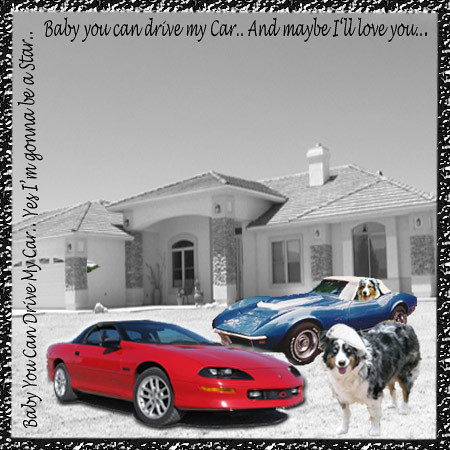This image is a square, black-and-white photograph framed like an old composition copybook. It features a suburban house with three large windows and a garage, and an ornate entryway. Superimposed in color on the grayscale background are two American sports cars: a red Camaro in front and a blue early-1970s Corvette with a white top behind it. In front of the blue Corvette stands a dog, either a Collie or an Australian Shepherd. Another dog of the same breed appears to be in the driver's seat of the blue Corvette. The photo is bordered with cursive text; along the top, it reads: "Baby, you can drive my car, and maybe I'll love you," and along the left side: "Baby, you can drive my car, yes, I'm going to be a star."